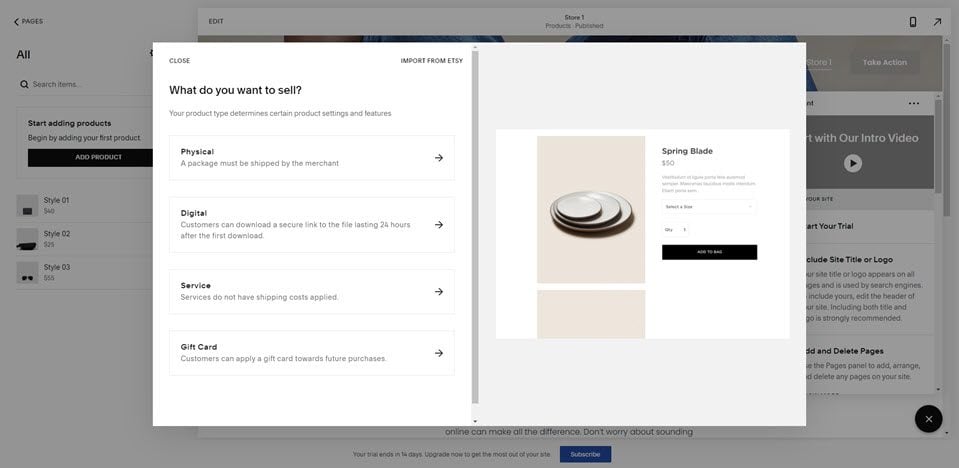The image appears to be a screenshot from a website, possibly similar to platforms like Etsy or a marketplace for selling luxury used goods. In the background, there's a standard webpage layout where users can browse or shop for various items and services. Superimposed on this background is a prominent pop-up dialog box asking, "What do you want to sell?" The options listed in the pop-up include Physical, Digital, Service, Gift Card, and Spring Blade, although the last option is not very clear. In the upper left corner of the pop-up, there's a "Close" button, allowing users to exit the prompt if they change their mind. The image emphasizes the platform's diverse selling options, accommodating anything from physical products to digital services, gift cards, and potentially even specialized items.